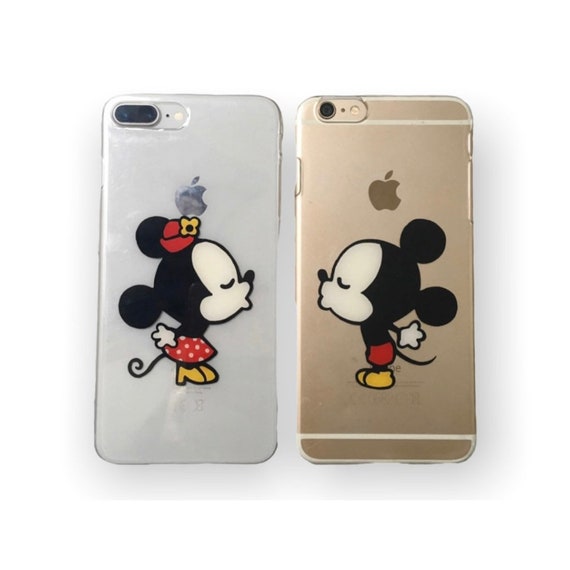The image depicts two Apple iPhones with decorative plastic back covers featuring Mickey and Minnie Mouse in a kissing pose. The phone on the left has a metallic grey cover with Minnie Mouse facing right, eyes closed, leaning in to kiss Mickey. The phone on the right sports a metallic brown cover with Mickey Mouse facing left, also with eyes closed, leaning in towards Minnie. Both characters are illustrated in vibrant colors, including black, white, red, and yellow. The background of the image is a light green color, providing a soft contrast to the metallic tones of the phone cases. There is no text on the picture, emphasizing the visual appeal of the scene. The overall style is playful and charming, capturing a romantic moment between the beloved Disney characters.